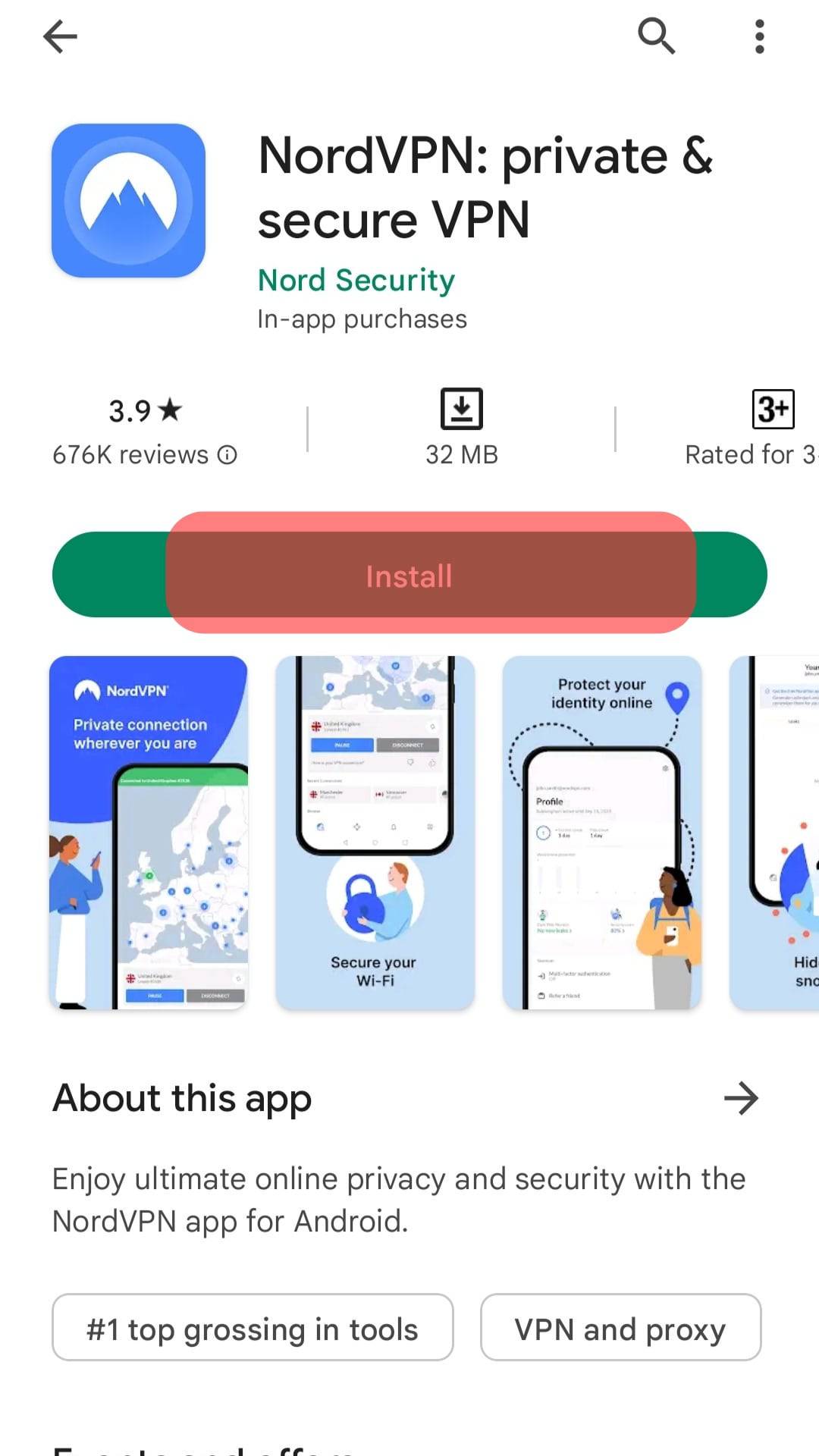The image is a screenshot of an app download page in an app store for the application "NordVPN." At the top, the app name "NordVPN: Private & Secure VPN" is displayed prominently. To the left of the app name, there is a blue square icon featuring a white background with an illustration of a mountain. Below the title, in green text, it reads "Nord Security," indicating the app developer. Directly beneath that, in black text, it notes "In-app purchases."

On the left side of the interface, the app's rating is shown as 3.9 stars, based on 676K reviews. Positioned centrally, there's a download button indicating the app size of 32 MB. On the right, the age rating is displayed as "3+," meaning the app is suitable for users aged 3 and up.

Below these details, there is a hunter green "Install" button with white text. There is also a noticeable translucent red rectangle partially surrounding the inner area of the "Install" button, highlighting it.